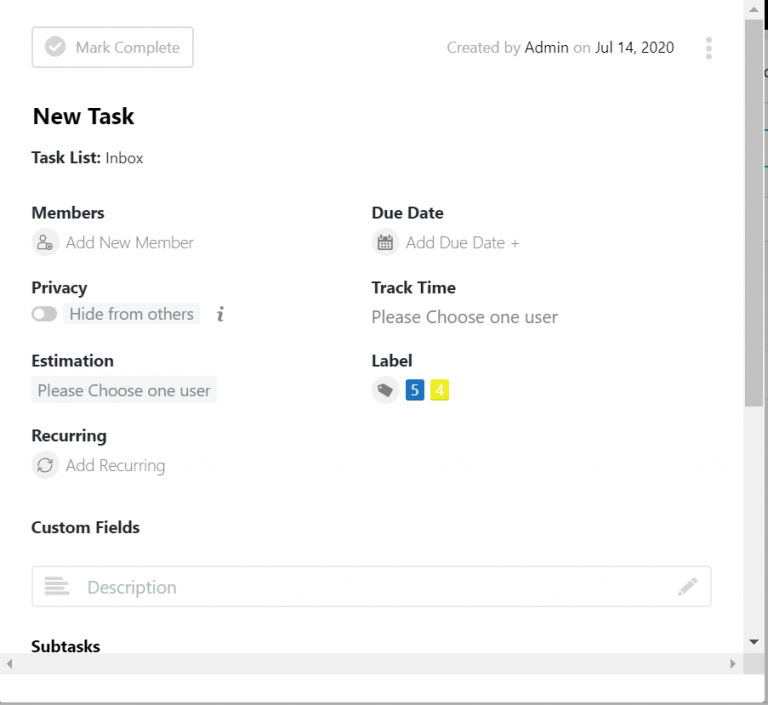Screenshot Description:

The image is a screenshot of a task management page against a white background, with the text predominantly in dark black print. Featured at the top is a watermark section bordered and labeled "Mark Complete," accompanied by a grayed-out circle containing a checkmark. Beneath this section, it is noted that the task was created by 'admin' on July 14, 2020.

The main body of the page begins with the heading "New Task" in bold font. Below this, there are several fields and functionalities laid out:

1. **Task List**: A boxed area intended for entering or selecting the task list.
2. **Members**: Displays an icon representing a member, alongside an option labeled "Add New Member".
3. **Due Date**: Includes a calendar icon with a prompt to "Add Due Date".
4. **Privacy**: Features a toggle button marked "Hide from Others".
5. **Track Time**: Requests user selection with the phrase "Please choose one user."
6. **Estimation**: Boldly presented term asking to "Please choose one user."
7. **Label**: Displays multiple small label icons for classification or tagging purposes.
8. **Recurring Tasks**: Depicted with an infinity symbol and labeled "Add Recurring".
9. **Custom Fields**: A section for additional, user-defined fields.
10. **Description**: An area designated for detailing the task.
11. **Subtask**: A section to list out any sub-tasks.

On the right side of the page, there is a vertical scroll bar indicating more content might be visible upon scrolling down.